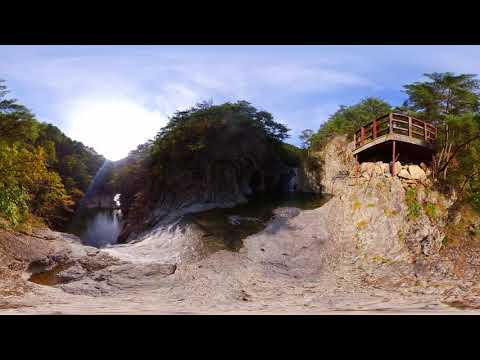This panoramic photograph captures a beautiful natural scene featuring a tranquil lake or pond with a wooden patio perched atop a rocky outcrop. The image reveals a 360-degree view, appearing slightly warped, that showcases both the foreground and background. To the right side, the wooden patio, partially painted white and supported by a single pillar embedded in the rock, stands on a small cliff surrounded by trees. The left side of the image displays a river with white rapids, tumbling over dark rocks, with lush green trees flanking both sides. The sky above is a mix of blue with patches of clouds, and the sun’s glare is visible, casting a soft glow over the trees. The photograph is encapsulated by a thick black border on the top and bottom, adding a framed effect to this picturesque landscape.